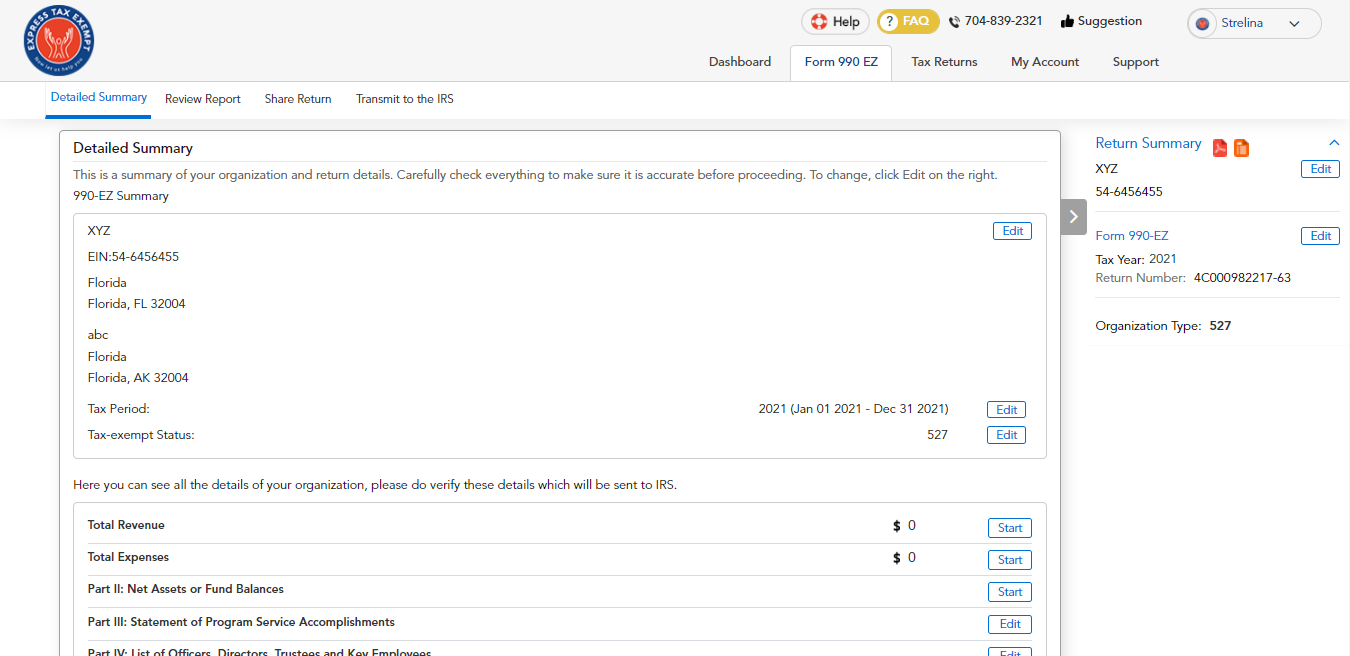In the image, the logo for ExpressTaxExempt is prominently featured in the top left corner. Various categories are displayed, including "Dashboard," "Detailed Summary," "Review Report," "Share Return," "Transmit to the IRS," "Form 990-EZ," "Tax Returns," "My Account," "Support," "Help," and "Frequently Asked Questions." There's also a section for "Suggestions" and a prominently displayed phone number.

Focusing on the "Detailed Summary" section, this area provides an overview of the organization and return details. Users are advised to thoroughly review this information for accuracy, and if any changes are needed, they can click the "Edit" button on the right-hand side. The summary of Form 990-EZ is shown, with fields such as "Total Revenue" and "Total Expenses" both listed as $0. Additionally, Part 2 emphasizes "Net Assets or Fund Balances," and Part 3 highlights the "Statement of Program Service Accomplishments." A list of offices, directors, trustees, and key employees is also included in this detailed summary.